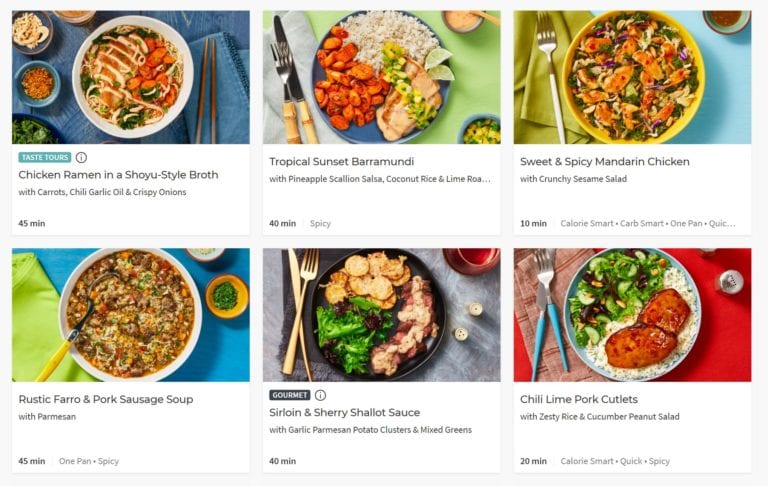This collection features a tantalizing array of culinary delights presented in a sequence of immaculate images. Each photograph captures a beautifully plated dish, meticulously detailed below:

**First Row:**
1. **Chicken Ramen in Shoyu Style Broth**
   - Description: A comforting bowl of chicken ramen served in a richly flavored shoyu broth, accompanied by tender carrots, a drizzle of chili garlic oil, and topped with crispy onions. Perfect for a gourmet tour, this dish promises a journey of taste in just 45 minutes.
   
2. **Tropical Sunset Bar Monday**
   - Description: An exotic plate featuring sweet and spicy mandarin chicken, complemented by a vibrant pineapple and scallion salsa, coconut-infused rice, and garnished with a lime wedge. The dish is paired with a crunchy sesame salad, offering a harmonious blend of flavors and textures.

**Second Row:**
1. **Rustic Farro and Pork Sausage Soup**
   - Description: An inviting, hearty soup made with farro and succulent pork sausage, enriched with the sharp, salty taste of parmesan. This rustic dish is ideal for those seeking comfort food with a touch of elegance.

2. **Sirloin with Sherry Shallot Sauce**
   - Description: A gourmet plate featuring tender sirloin steak drizzled with a luxurious sherry shallot sauce. The meal is beautifully accompanied by garlic parmesan potato clusters and a fresh mixed greens salad, making it a refined yet hearty option.

3. **Chili Lime Pork Cutlets**
   - Description: Quick and calorie-smart, these zesty chili lime pork cutlets are served with vibrant rice and a refreshing cucumber peanut sauce. This dish is a spicy and speedy choice, perfect for a flavorful meal in just 20 minutes.

Each image showcases the food atop a well-set table, with a diverse palette of colors including blue, yellow, green, red, gray, orange, silver, black, and white, enhancing the visual appeal of the dishes. The vibrant settings and artistic presentation reflect meticulous attention to detail, adding to the overall allure of this gastronomic presentation.